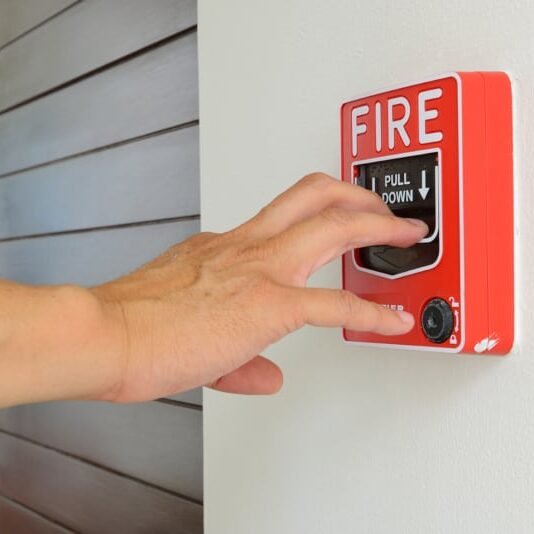The image shows a white individual's hand activating a red fire emergency device mounted on a white wall. The device prominently displays the word "FIRE" in white letters, with a black handle labeled "PULL DOWN" that is being pulled by the person's hand, likely triggering the alarm. There is a black, oval-shaped speaker on the box, and a small keyhole in the bottom right corner for locking or unlocking the device. In the background, the left side of the wall features gray, possibly wooden or metal, horizontal slats, adding to the composition's detail. The scene appears to be set in a professional environment, such as a business or office building.